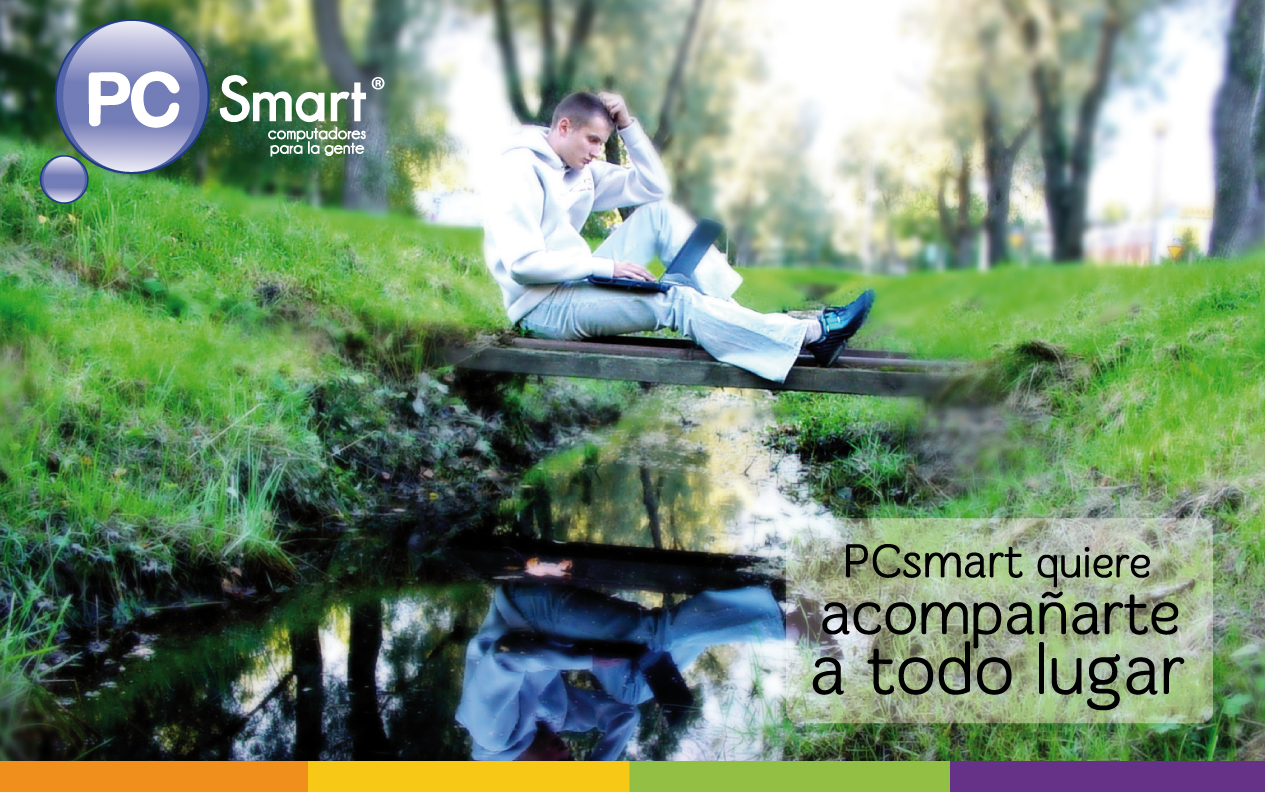This image, likely an advertisement, features a Caucasian man sitting on a small wooden bridge spanning a creek in a lush, green meadow. The bridge, approximately six feet long, sits in a park-like setting, bordered by grassy fields and flanked by trees on either side. The man, dressed entirely in white with black shoes, is wearing a long-sleeved hoodie and white pants. He adopts a relaxed pose with one leg up, elbow resting on his knee, and his hand placed casually on his head. In his other hand, he holds a laptop on his lap. 

In the upper left corner of the image, there's a purple circle with "PC" written in white letters next to the word "Smart," supported by the tagline "Computadores para gente" (computers for people in Spanish). The bottom right corner features a similar phrase, "PC Smart quiere acompañarte a todo lugar" (PC Smart wants to accompany you everywhere). Additionally, the image's bottom section is accentuated with an orange, yellow, green, and purple bar, enhancing the advertisement’s colorful and engaging nature.